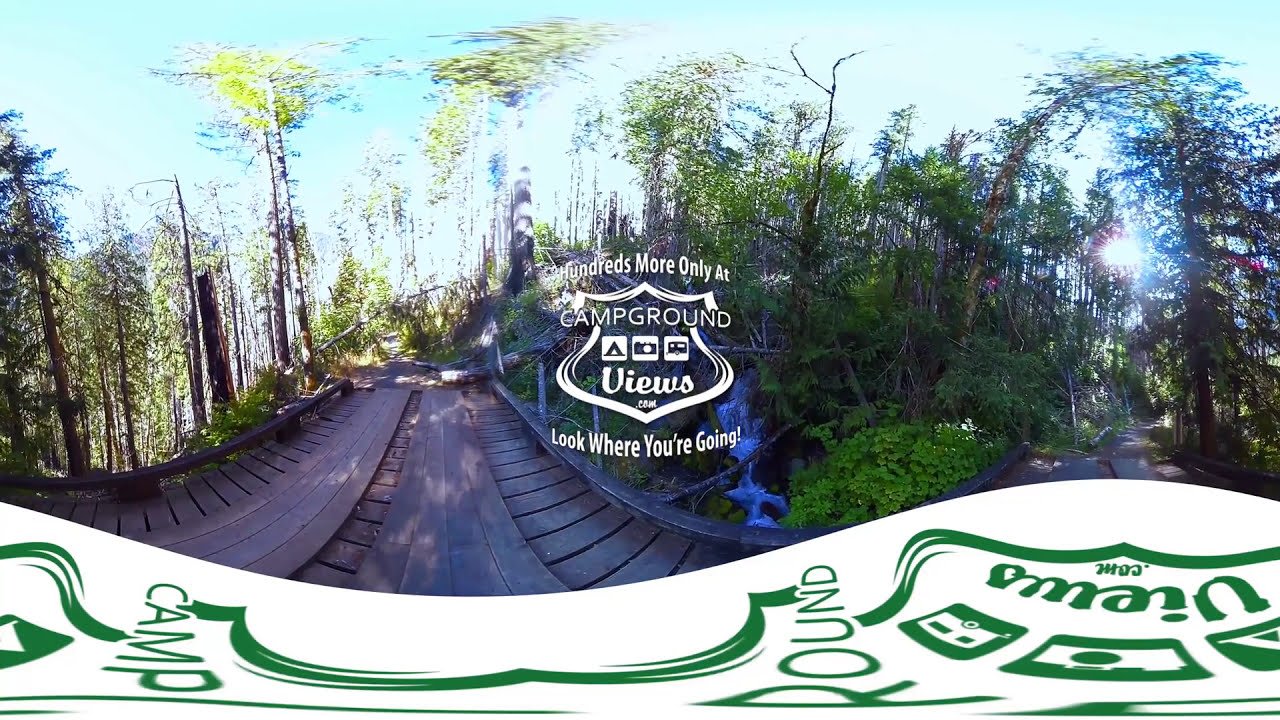This panoramic outdoor 360-degree image captures a scenic wooden boardwalk winding through a densely vegetated area. The boardwalk, curving around and meeting in the center, is flanked by narrow, standing trees and lush leafy vegetation, including creeping ground cover that adds to the scenic beauty. The ground slopes steeply away from the boardwalk on both sides, creating a sense of depth and perspective. A prominent curved white band at the bottom of the image displays the word “camp” in green print, potentially part of a graphic superimposed onto the photograph rather than an actual object. Overlay text in the photograph reads "hundreds more only at campgroundviews.com," suggesting this might be part of a campground advertisement. The clear blue sky peeks through the canopy, adding a tranquil, natural ambiance. Overall, the image has a somewhat wavy and surreal quality, characteristic of 360-degree or virtual reality imaging, giving the vegetation and boardwalk a dreamy, swaying appearance.